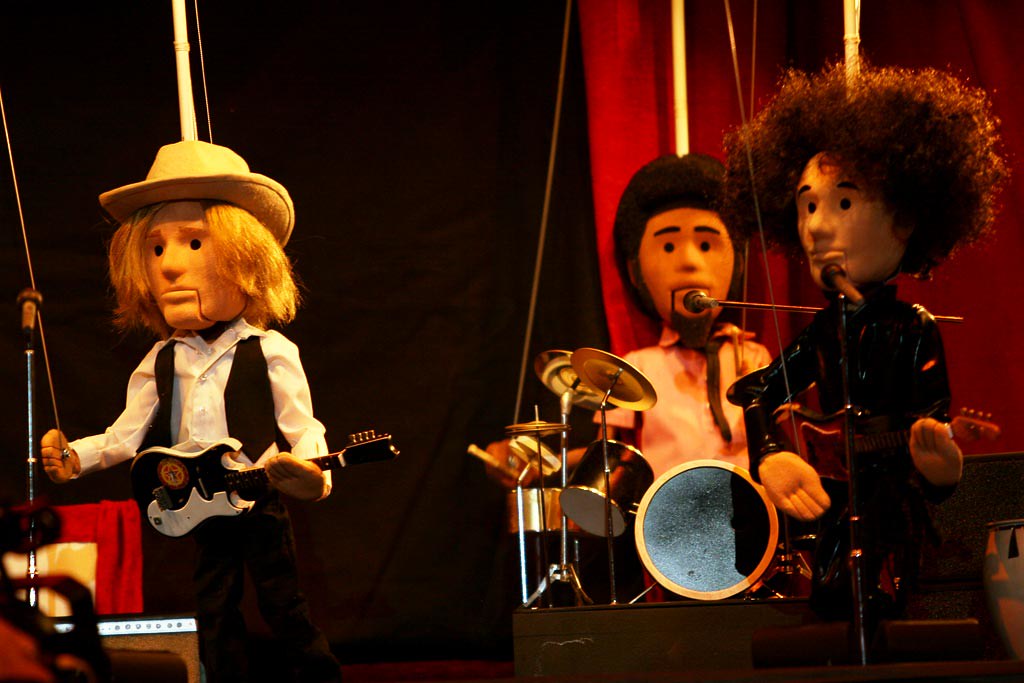The image depicts a band of three marionette musicians set against a backdrop featuring a black and a red curtain. On the left, a marionette with long blonde hair under a cowboy hat is dressed in a white shirt and brown vest, playing a black and white guitar. The strings attaching to his arms and legs are clearly visible. To the right, another marionette guitarist sports big bushy brown hair, almost like an afro, and is clad in a dark outfit. In the background, a drummer marionette with short dark hair and a goatee is seated behind a complete drum set with cymbals, a snare drum, and other drums. The strings and attachments that connect these puppets to the puppet master are also clearly visible, adding an authentic touch to this detailed and vivid depiction of a marionette band.